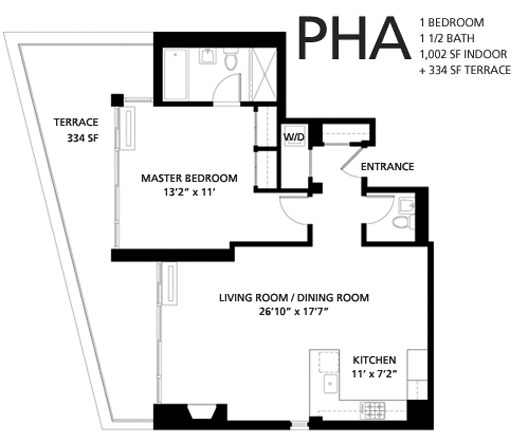The blueprint of the apartment, labeled "PHA" in large text on the top right corner, showcases a detailed layout of the unit. It is described as a one-bedroom residence with one and a half bathrooms, covering a total of 1002 square feet indoors, along with an additional 334 square feet terrace. The blueprint provides a top-down view of the apartment's arrangement.

To the left of the blueprint, there is a uniquely shaped, almost triangular terrace. To the right of the terrace, centrally located within the layout, is the master bedroom. The master bedroom's dimensions are specified to be 13.2 feet by 11 feet. Adjacent to the master bedroom is a designated area for a washer and dryer, close to the entrance of the apartment. Below the master bedroom, the blueprint illustrates the living room, which seamlessly transitions into the kitchen area situated at the bottom right of the living room. Each room is meticulously drawn, providing a comprehensive visualization of the apartment’s spatial organization.